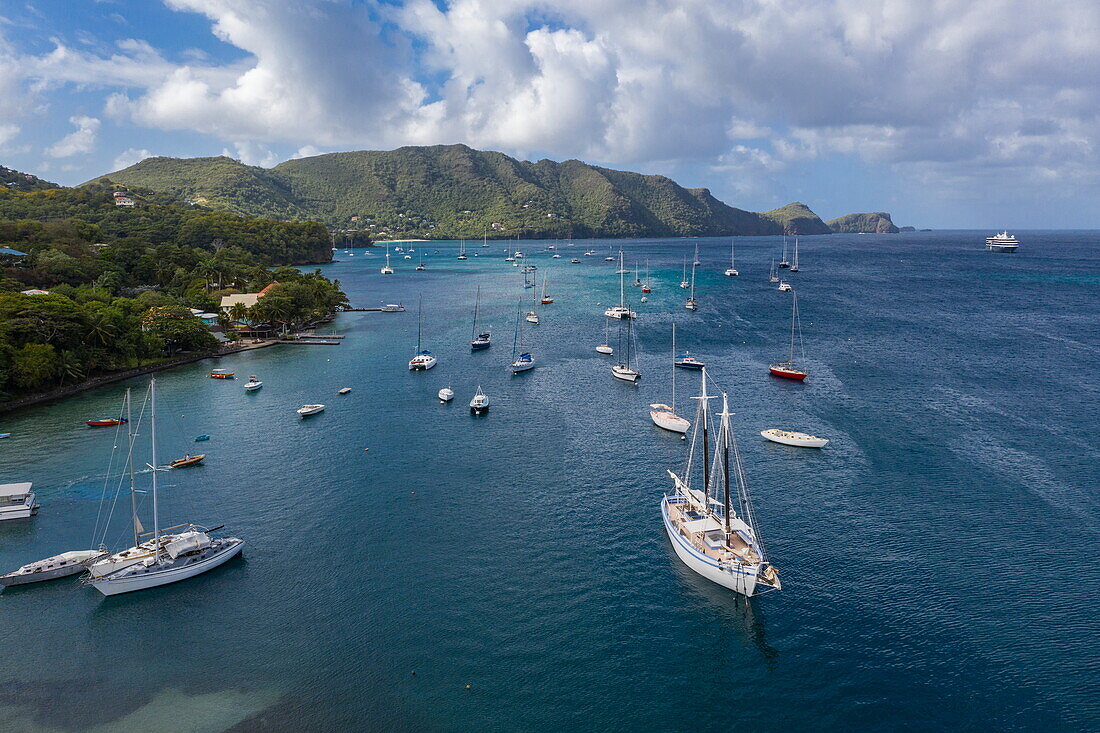This image captures a vibrant scene on a bright sunny day, showcasing a large, clear blue body of water, possibly an ocean or bay. The water, rich and pristine, is teeming with over fifty boats of varying sizes, predominantly white, but also featuring accents of blue, red, and orange. Most boats are oriented in the same direction, suggesting a forward movement toward the horizon. Amidst the fleet, a notable outlier boats is situated further to the right, appearing larger than the others. 

The left side of the image reveals lush, green terrain with dense vegetation and scattered houses nestled among trees. Extending from this verdant land are docks jutting out into the water, along with glimpses of palm trees and other structures. The far horizon is marked by more mountainous, green areas, enhancing the image's natural beauty. The sky above is a clear blue interspersed with picturesque clouds, emphasizing the tranquil, yet lively nature of the scene.